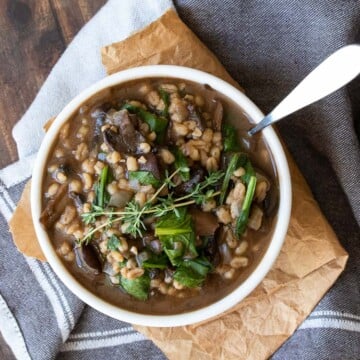This image shows a detailed, top-down view of a hearty bowl of soup in a white-rimmed bowl, complemented by a silver spoon with the handle protruding from the upper right corner. The soup itself has a rich brown broth, indicative of brown gravy, and contains an assortment of ingredients including white beans (possibly white kidney beans), barley, whole spinach leaves, small potatoes or quinoa seeds, mushrooms, and what appears to be pieces of beef. The presentation is rustic, with a folded paper bag placed directly under the bowl. Beneath the paper bag lies a gray cloth with white stripes, and part of a brown wooden tabletop is visible in the image's upper left corner. The scene evokes a cozy, home-cooked meal ambiance.